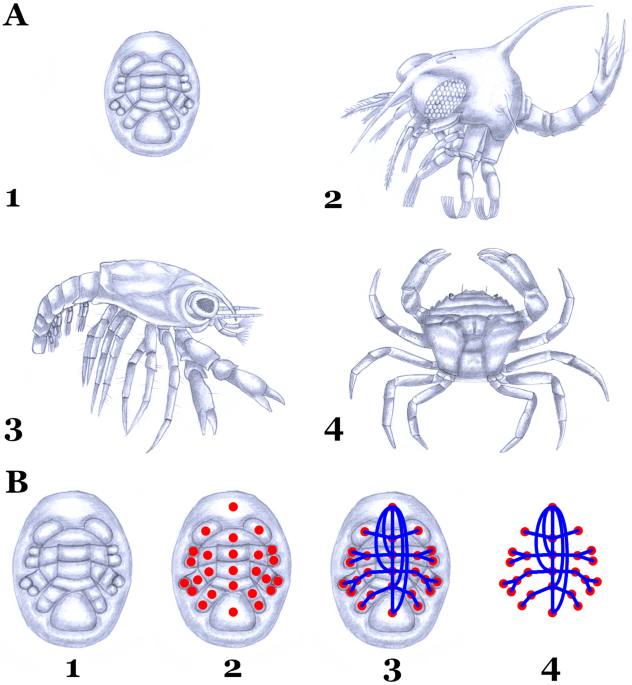The image is a detailed scientific diagram featuring illustrations of various crustaceans and sea creatures. The layout is divided into two main sections labeled "A" at the top and "B" at the bottom, each comprising four images rendered in a gray and white pencil-shaded style.

**Section A:**
- **A:** Depicts the body or abdomen section of a larva-like creature.
- **A1:** Shows a shrimp-like crustacean with claws facing right.
- **A2:** Illustrates a creature resembling a mutated combination of a fly, lobster, and shrimp, with large compound eyes, facing left.
- **A3:** Features a hybrid appearance, somewhat like a shrimp and lobster combined.
- **A4:** Represents a regular crab, which could be a blue crab or stone crab.

**Section B:**
- **B1:** Portrays the same body section as the larva in image A, but without legs.
- **B2:** Adds red dots over the body section, indicating specific points, possibly anatomical landmarks.
- **B3:** Connects the red dots with blue lines, forming a network, potentially representing veins or nerves.
- **B4:** Removes the body section entirely, leaving only the red dots and the blue connecting lines, illustrating a simplified framework of the anatomical connections.

The detailed and systematic depiction highlights the anatomy and possible internal structures of the crustaceans, showcasing developmental stages or anatomical studies relevant to biological and anatomical education.